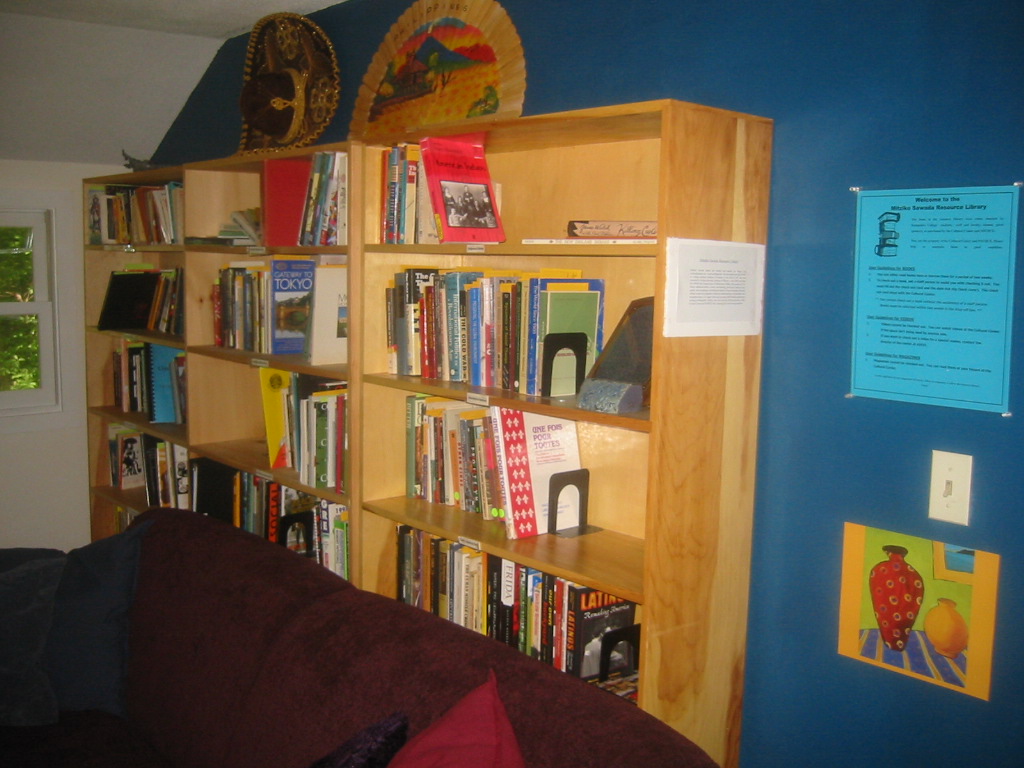The photograph captures a cozy and well-decorated room with multiple elements of visual interest. Against a blue-painted wall, there are three light wood bookshelves filled with an array of hardcover books, some of which are non-fiction titles about Tokyo and Latina culture. Atop these bookcases rest an ornate brown fan featuring a desert scene, and a brown and gold sombrero, both leaning against the wall. To the right of the bookshelves, a blue poster with various lines of black text hangs above a white light switch, which is currently in the off position. Below the light switch, there is a painting depicting two vases on a blue and yellow striped surface. In front of the bookcases, a brown fabric couch occupies the space, adorned with a red cushion on one side and a black cushion on the other. A white wall to the left features a double-pane window with white trim, offering a glimpse of green leaves outside. This room combines elements of homey comfort with a sense of scholarly organization.